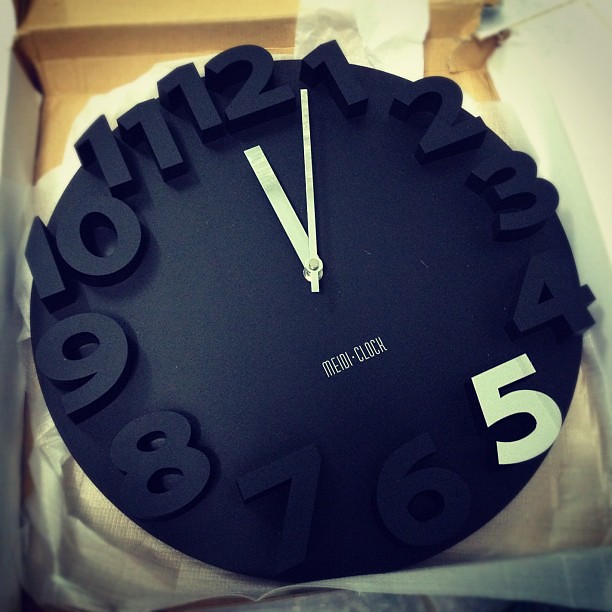This photo features a stylish clock with a slightly tilted black textured face. The clock's numbers are embossed and appear thicker than the clock’s surface, either in a dark blue or deep black similar to the face itself, with the exception of the number five, which stands out in bright white as though it were drawn or photoshopped on. The clock hands are stark white, with the hour hand as a thick rectangle and the minute hand a longer, thinner rectangle, indicating the time as 12:04. Below the center of the face, the brand name "M-E-I-D-I dot clock" is displayed in gold. The clock is situated in a partially open cardboard box, revealing clear transparent wrapping paper behind it.